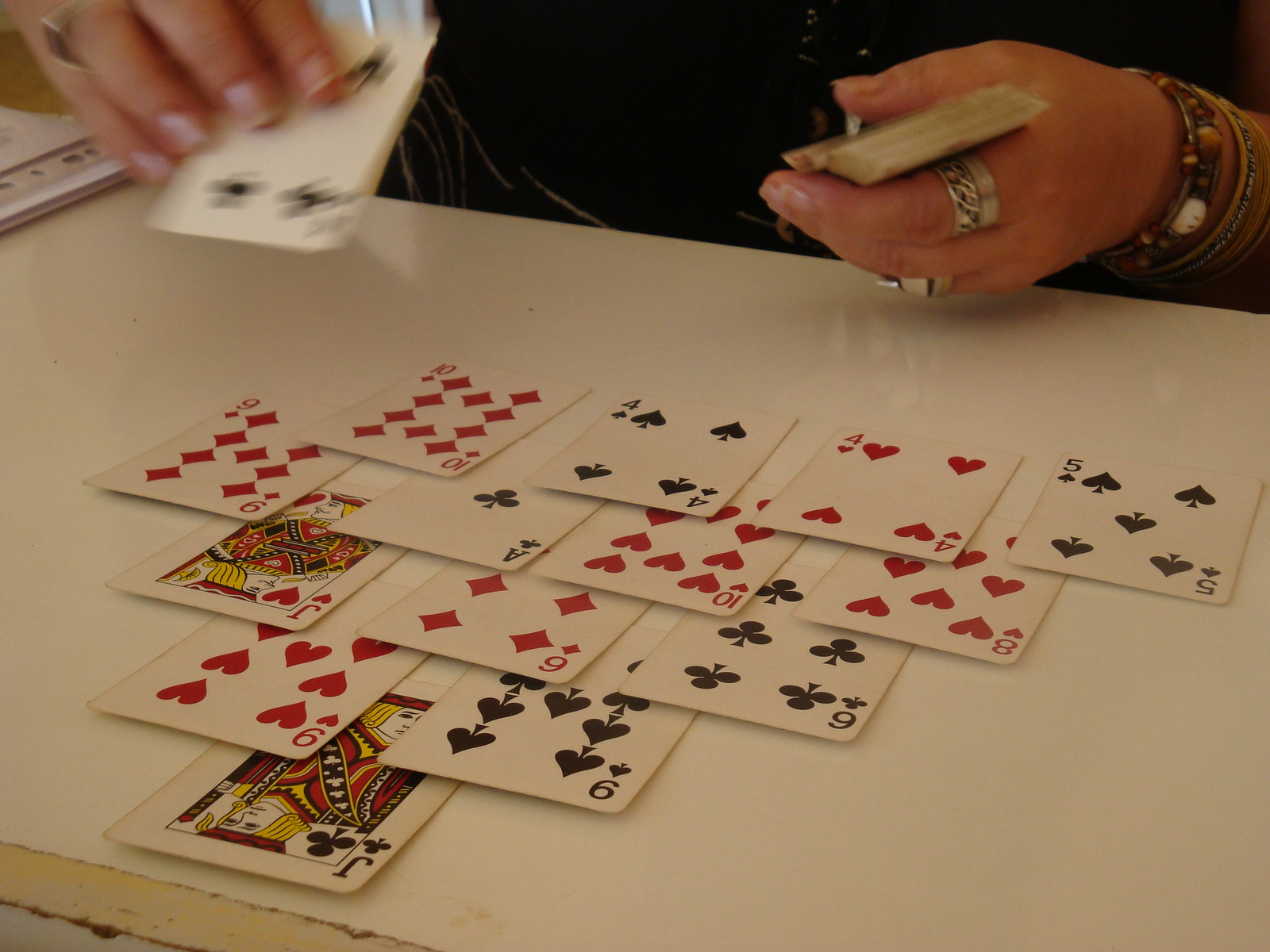A person is meticulously dealing playing cards on a white, possibly runner-covered, table. The cards are arranged in a preliminary pyramid layout, all face up to reveal their suits and numbers. At the apex sits a jack of clubs. In the second row are a nine of spades and a nine of hearts. The third row consists of a six of clubs, a six of diamonds, and a jack of hearts. The fourth row features an eight of hearts, a ten of hearts, an ace of clubs, and a nine of diamonds. In the final row, a five of spades, a four of hearts, a four of spades, and a ten of diamonds are newly joined by a four of clubs, which is currently being placed. The dealer, wearing two prominent rings and a large-beaded bracelet on their left hand, deftly pulls cards from the deck held in that hand to lay them out with their right hand. The table, with its shiny white surface, is topped by a cream-colored edge visible in the foreground, suggesting the white surface is an overlay or decorative runner.